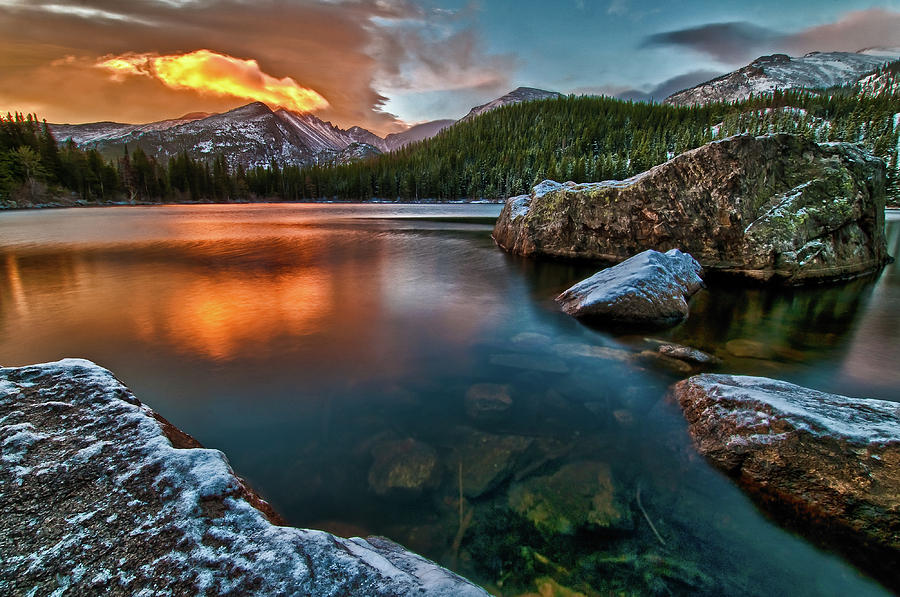In this breathtaking mountain landscape captured at sunset, the scene unfolds with an impressive display of nature's beauty. In the foreground, there are two massive snow-covered rocks on the left and right sides of the image, framing a smaller, similarly snow-capped rock between them. The rocks are intricately detailed, showcasing every bump and cranny. Nestled amidst these colossal formations is a clear, serene pond that branches out and reflects the stunning colors of the sky. The water is incredibly transparent, revealing a bed of large brown rocks and casting pinkish and white reflections where the clouds cast shadows.

Beyond the pond, a dense line of green trees stretches across the width of the image, standing in stark contrast to the towering snow-capped mountains in the distance. The sky above is divided dramatically: on the right, it is a deep blue with streaks of grayish-purple clouds, while on the left, it presents a captivating gradient of brownish hues with openings of vibrant orange and yellow light from the setting sun. This light not only illuminates the sky but also casts a radiant glow across the surface of the pond, creating a mirror-like reflection of the sunset. The vivid colors and reflections, combined with the stillness of the water and the rugged grandeur of the rocks and mountains, evoke a profound sense of isolation, beauty, and tranquility.